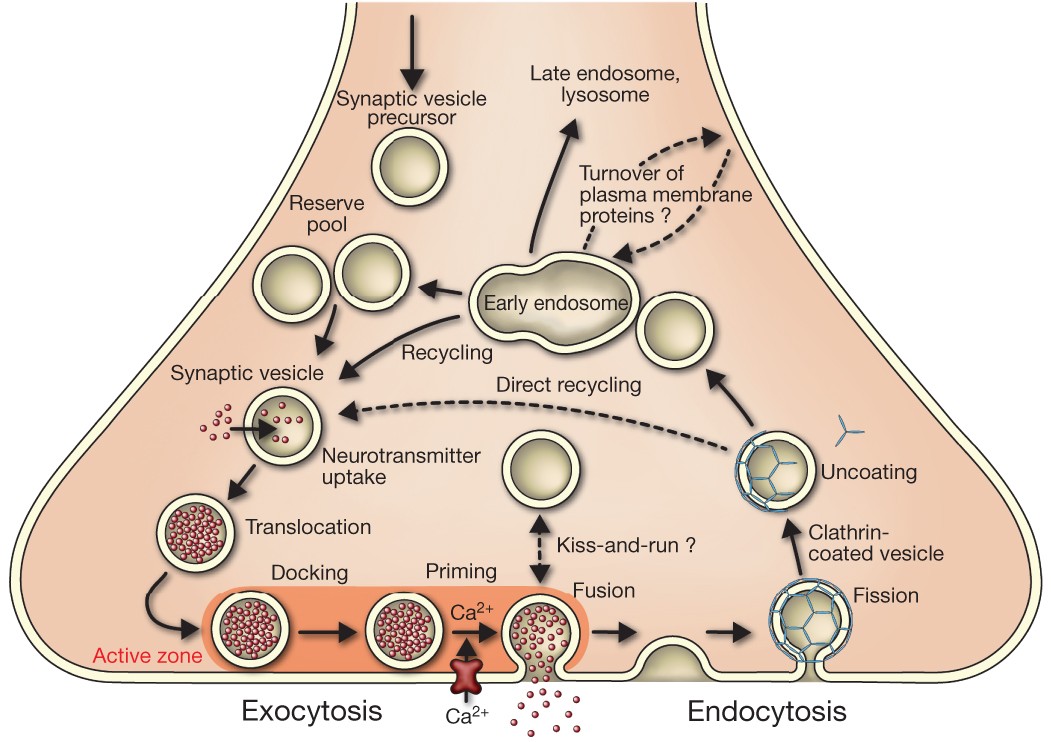This detailed scientific diagram illustrates the complex life cycle of synaptic vesicles within a neuron, represented by a rounded triangular shape with a pale peach interior and off-white cream borders. Starting from the top with a downward arrow, it depicts the progression from synaptic vesicle precursors to reserve pools. The synaptic vesicles, initially depicted as gold circles with a beige outline, transition through various stages including translocation, docking, and priming, indicated by arrows and textual annotations.

As the process moves into the active zone, highlighted in red text, the vesicles appear densely packed with small red dots, signifying neurotransmitter uptake. Following this, the vesicles undergo fusion, kiss and run, fission, and uncoating. Vesicles in the stages of fission and uncoating are shown with blue hexagonal patterns. The diagram further details the return journey of vesicles towards the early endosome.

Notably, the bottom left is labeled 'exocytosis,' and the right side 'endocytosis,' marking critical points of vesicle turnover and membrane recycling. The elements within the diagram are connected through a network of arrows and labeled with text such as "synaptic vesicle precursor," "reserve pool," "translocation," "docking," "priming," "fusion," "fission," "clathrin-coated vesicles," "uncoating," "early endosome," "recycling," "late endosome," "lysosome," and "turnover of plasma membrane proteins." The overall flow and interactions within this process are meticulously detailed, providing a comprehensive visual overview of synaptic vesicle dynamics.